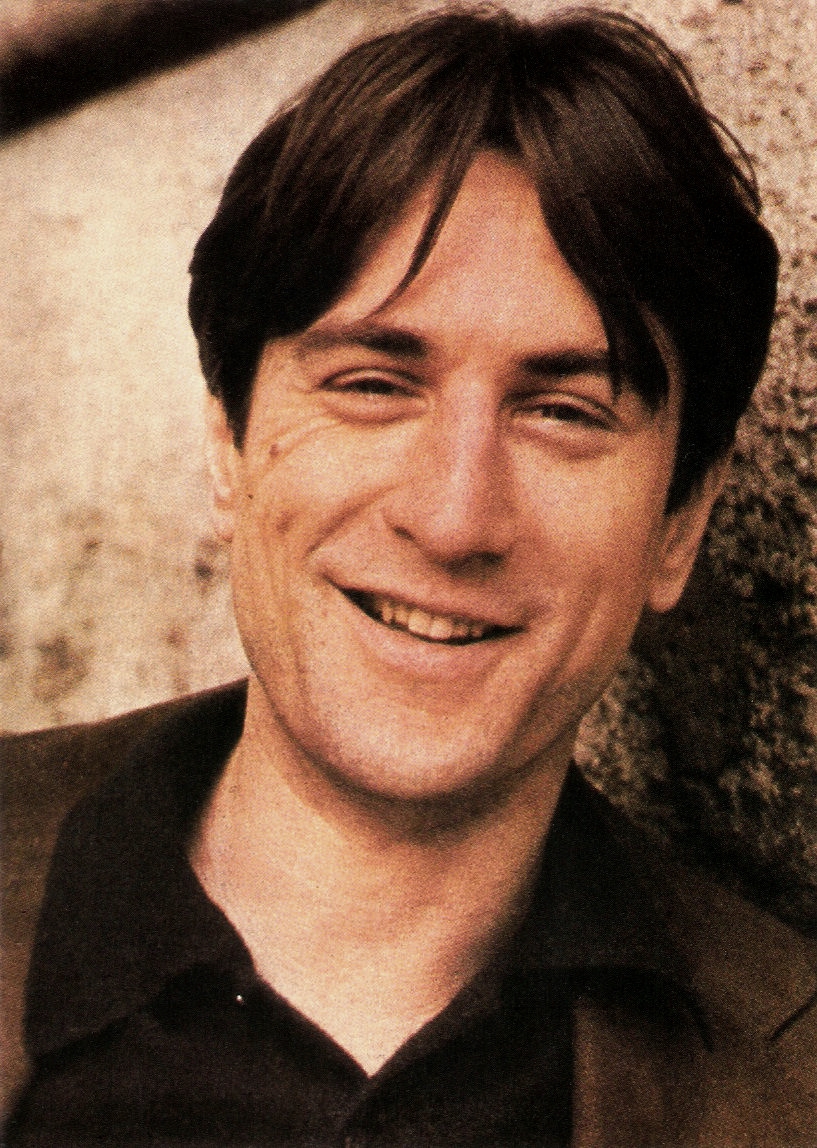This image features a very young Robert De Niro, likely in his mid-20s to early 30s, standing in front of a stone or concrete wall, likely taken in daylight with an overcast sky. His thick, dark hair is styled with pseudo bangs, and his vibrant brown eyes exude a lively energy. De Niro's distinguished smirk reveals his teeth and highlights the trademark mole on his right cheek. He has pronounced laugh lines and very thick, dark eyebrows. His complexion appears to be fair but with a notable Mediterranean, Italian-like look. He is dressed in a black button-down shirt and a brown coat, exuding a casual yet polished look that complements his young, confident demeanor. His head is slightly tilted to the side, striking a relaxed yet charismatic pose.